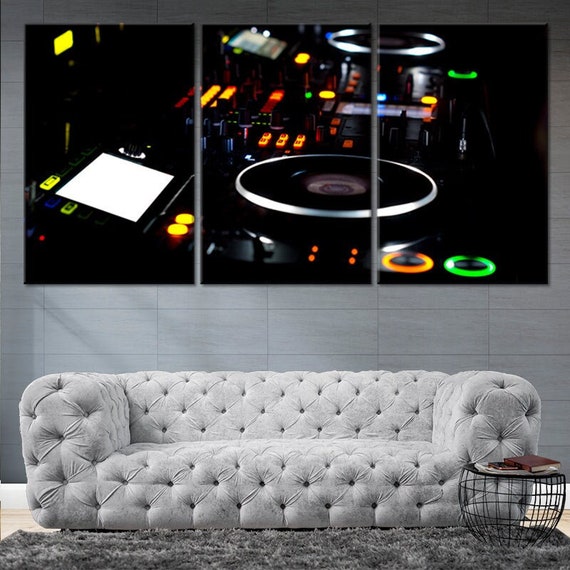The image depicts a modern living room with a minimalist yet cozy aesthetic. Dominating the foreground is a plush, light gray, tufted couch featuring a soft, buttoned design that gives it a slightly wrinkled appearance. Draped over the floor in front of the couch is a dark gray, shaggy rug that adds an element of texture to the setting. To the right side of the room, a round wire mesh side table sits adorned with a few dark brown books and a phone. The backdrop of the room is a striking gray wall decorated with a large, three-panel artwork that vividly captures a detailed close-up of a DJ setup, with visible buttons and spinners on dark backgrounds, giving the room a modern, edgy vibe.